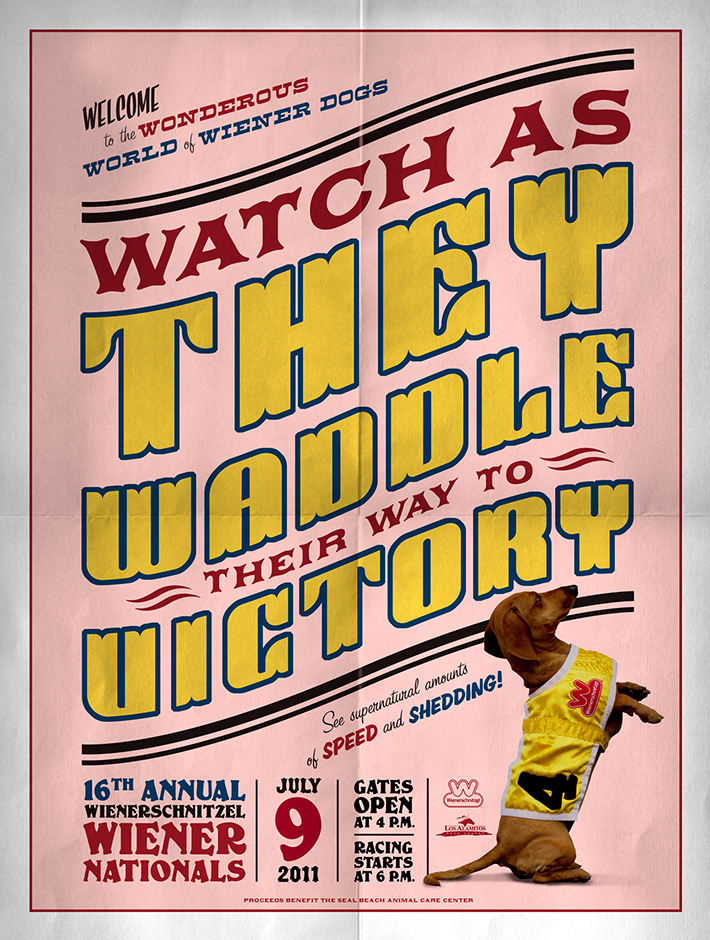The vertical poster features a silver frame, a white border, and a pink background. At the top, in playful towel-sized font, it reads, "Welcome to the wondrous world of wiener dogs," with "welcome" in black, "wondrous" in red, and "world of wiener dogs" in blue. Below, two curving black lines, one thin and one thicker, sweep up and to the right. The text beneath reads, "Watch as," in red capitals, "they waddle" in large yellow letters, "their way to" in small red font, and "victory" in large yellow letters. The same curved lines appear again. At the bottom, in blue, it announces "16th Annual," followed by black text, "Wiener Schnitzel," and red text, "Wiener Nationals." The date "July 9, 2011" is shown, with "July" in black, a large "9" in red, and "2011" in black. It notes that gates open at 4pm, with a line separating this from "racing starts at 6pm." The tagline reads, "See supernatural amounts of speed and shedding." In the bottom right corner, a brown wiener dog, smooth-coated and long with floppy ears, stands on its hind legs. It sports a yellow overcoat with the number 4, posed as if ready to race with its short legs and pointed snout.